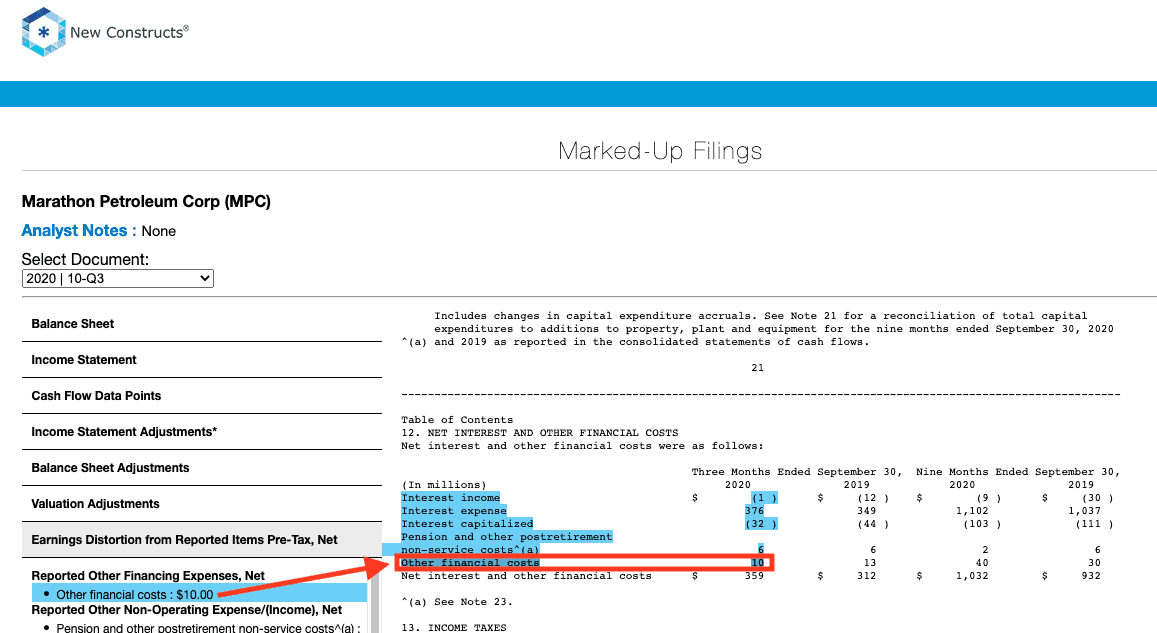In this screenshot of a financial analysis document, multiple sections provide detailed information regarding Marathon Petroleum Corporation's (MPC) financial filings. 

In the upper left corner, the label "New Construct" is displayed. Below it, the primary heading reads "Marked Up Filings." The left sidebar lists various menu options including "Balance Sheet," "Income Statement," "Cash Flow," "Data Point," "Income Statement Adjustment," "Balance Sheet Adjustment," "Valuation Adjustment," and "Distortion from Reported Items Pre-Tax Net."

One specific entry, highlighted in blue, indicates "Other Financial Costs: $10" which is noted to be reported as "Other Than Operating Expense or Income Net." This entry is additionally emphasized with a red arrow pointing to the main content area on the right.

At the top right corner, a note indicates "Includes changes in capital expenditure currency note 21 for reconciliation of total capital expenditures to additions to property, plant, and equipment." This note also mentions a time frame, "49 months ended September 30, 2020, and 2019," as reported in the "Consolidated Statement of Cash Flow."

Further down on the right, a section titled "Table of Contents" leads to "Net Result and Other Financial Cost," followed by a table comparing financial data across different periods. The columns are labeled "Three Months Ended September 30" and "Nine Months Ended September 30," displaying figures in millions. Categories include "Interest Income," "Interest Expense," "Interest Capitalized," "Pension and Other Retirement Non-Service Costs," and "Other Financial Cost." The specific entry "Other Financial Cost" is highlighted in blue and outlined in red, indicating its significance.

The meticulous composition of this document offers a granular view of Marathon Petroleum Corporation's financial adjustments and key metrics for the specified periods.